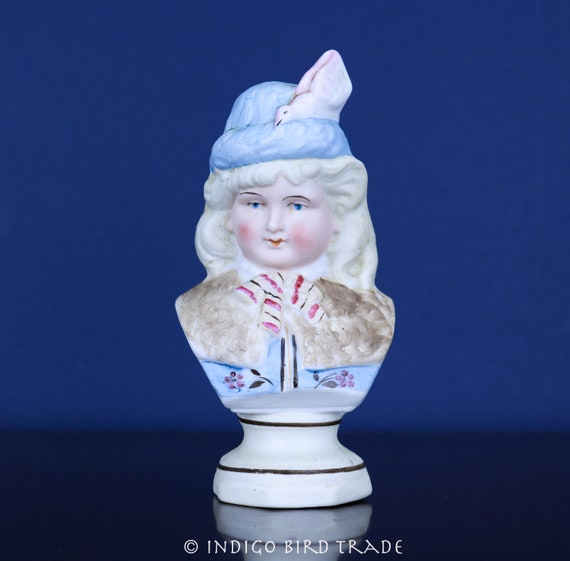This photograph showcases a detailed ceramic bust of a person characterized by several distinctive features. The sculpture, displayed on a dark blue reflective surface with a slightly lighter blue background, portrays the chest, shoulders, face, and head of the figure. The base of the bust is white, transitioning up to brownish fur over the shoulders. The person has long, curly white hair, red rosy cheeks, small red lips, and blue eyes. The head is adorned with a light blue, wool-style cap, upon which a small white bird is perched. The figure also appears to have a round face and is dressed in a brown jacket, detailed with a bow at the neck and a floral motif.